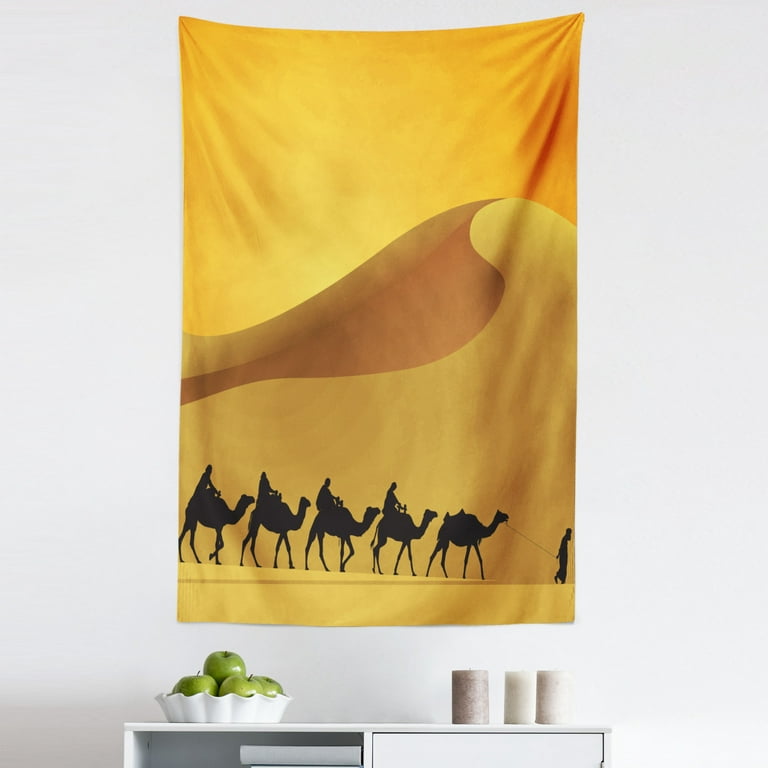In this detailed indoor photograph, a captivating scene is depicted within a white or slightly off-white room. A decorative towel, mimicking the hues of desert sands with gradients of yellows, tans, and dark browns, hangs on the wall. This towel features silhouettes of five camels walking in a line at the bottom, four of which have riders, while the front camel is being led by a person holding its reins. Below the towel is a white table or cabinet adorned with several items. On the right side of the surface are three off-white, chunky candles with shades of tan, while on the left, a white ceramic bowl holds several green apples. The minimalistic setup and precise elements create a serene and visually balanced composition.